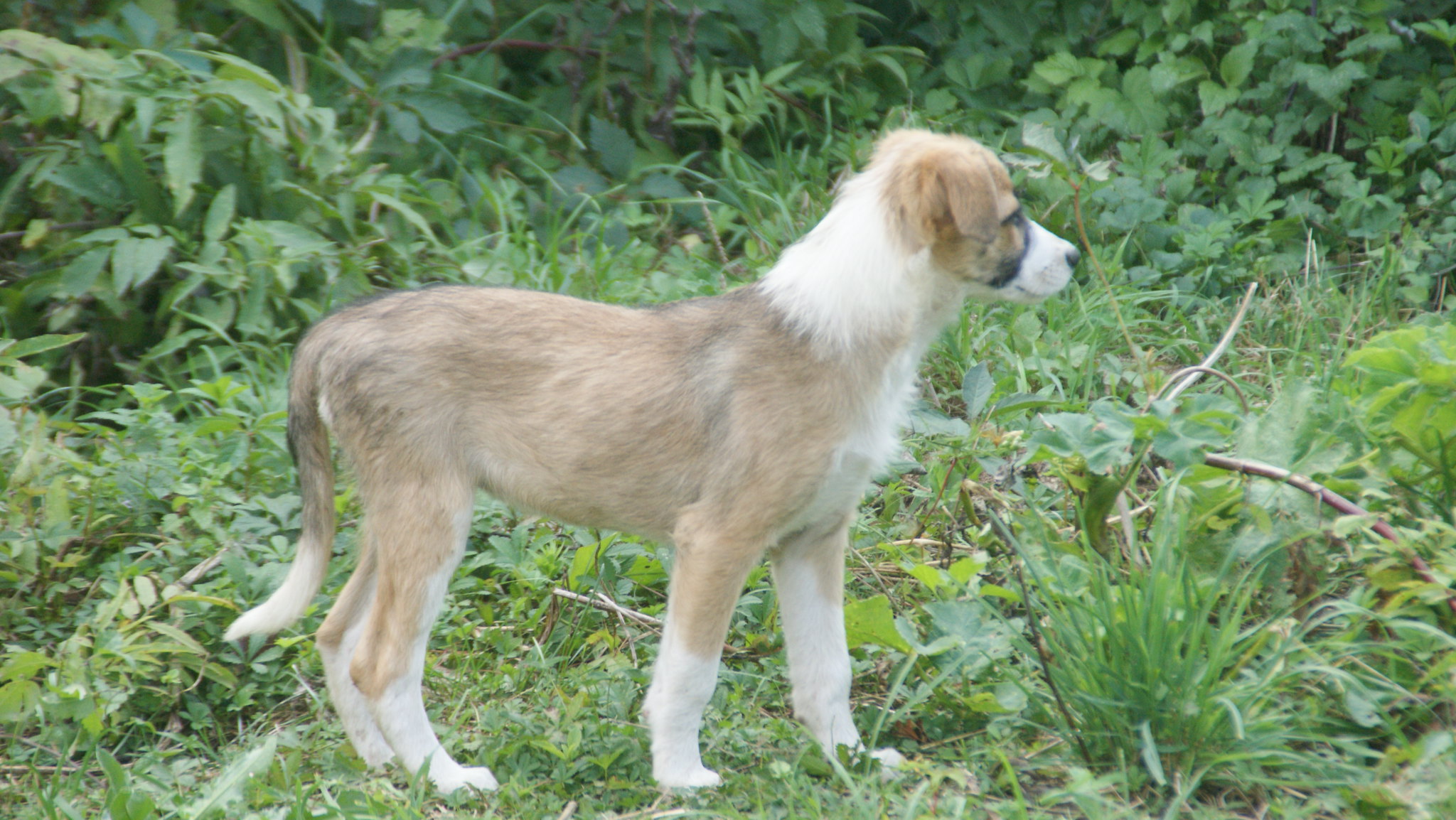A landscape-oriented photograph captures a young, cute puppy standing outdoors on a sunny day. The dog, which may be a shepherd mix, is centrally positioned in the image, standing on all four legs amidst a bed of grass and surrounded by green bushes and some sticks scattered on the ground. The puppy's coat is predominantly brown and black with distinctive white markings on its legs, the tip of its tail, neck, and muzzle. A notable black line separates the tan part of its face from the white muzzle. The dog is looking to the right, presenting a perfect profile with its floppy ears and tail relaxed down. The overall setting feels wooded and natural, emphasizing the puppy's attentive and curious demeanor.